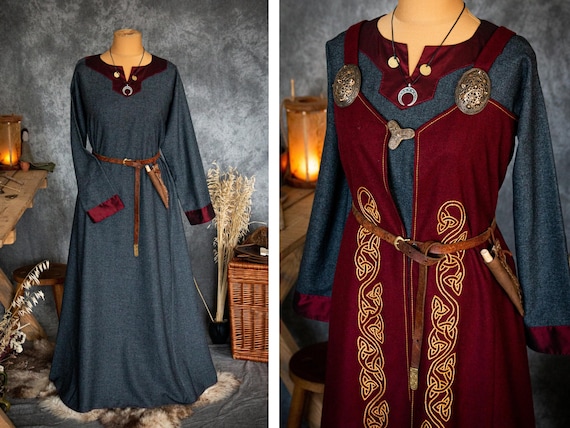The images depict two side-by-side photographs showcasing a detailed medieval-inspired outfit on a mannequin. In the left photograph, the garment is a long blue dress with long sleeves adorned with shiny burgundy bands at the edges and around the collar. The dress is cinched with a leather belt that includes a knife sheath. Around the mannequin's neck is a silver crescent moon necklace. The right photograph displays the same blue dress, now partially covered by an additional burgundy garment with gold trim running down the front. This over-layer features two silver buckles that secure the bodice with straps. The detailed setup also includes scene-setting elements such as a table and wheat, enhancing the historical ambiance.